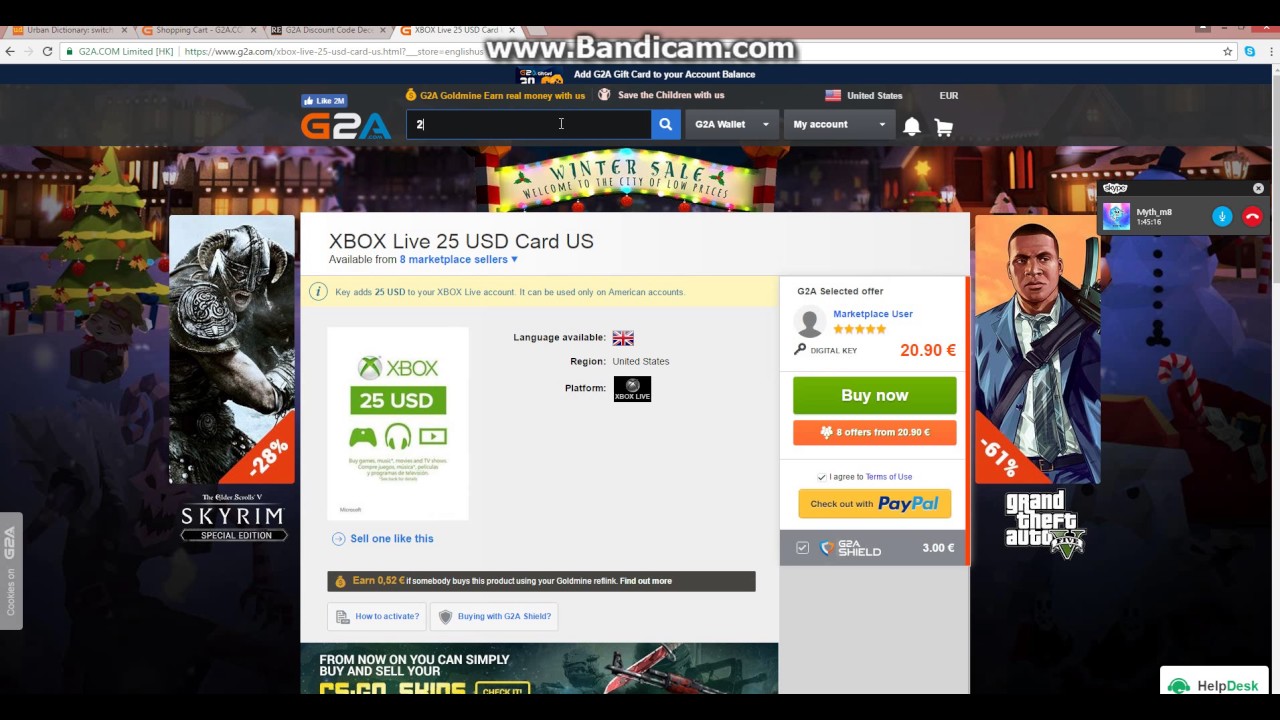Screenshot of a browser window, most likely either Microsoft Edge or Google Chrome. At the top, in large, bold letters with a grey shadow, the URL reads www.bandicam.com. There are four open tabs, with their titles too small to clearly discern. The visible text on the tabs suggests they are "Urban Dictionary," "Shopping Cart," some sort of "Discount Code" page, and an "Xbox Live" tab.

The highlighted tab is displaying a webpage on G2A's Bandicam site, specifically for purchasing an Xbox Live gift card worth 25 USD. The detailed description on the page indicates that the card adds $25 to an Xbox Live account and is only usable on American accounts. It includes information on language (American English), region (United States), and platform (Xbox Live). On the right side of the page, there’s a “G2A Selected Offer” from a marketplace user, pricing the card at €20.9 with a "Buy Now" option. There's also an option to pay via PayPal.